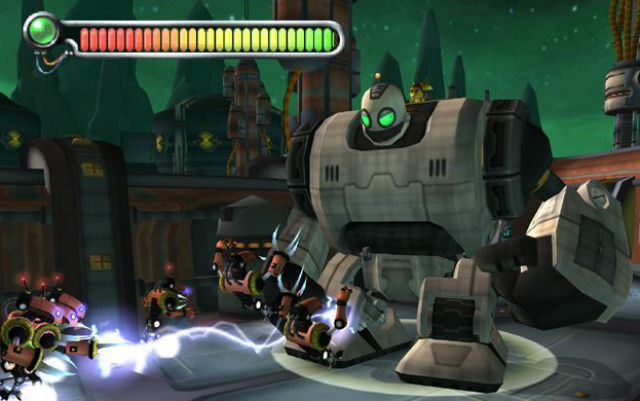This computer-generated image appears to be a scene from a video game, as indicated by the energy bar at the top of the screen. The energy bar, which is encased in a silver frame and includes a green circle on the left, transitions in color from red to yellow to green, suggesting it is fully charged.

Central to the scene is a towering, formidable robot occupying the right half of the image. This robot is crafted in silver and black, featuring a massive chest, powerful arms, and sturdy legs. Its small head, distinguished by a black mouth and black circles around its glowing green eyes, gives it a menacing appearance. 

In the foreground, several small red and yellow robots can be seen, emanating bolt-like sparks. It seems that the giant robot has just delivered a powerful kick to a couple of these smaller robots, sending them flying. 

The backdrop features a chaotic battleground, dominated by earthy brown tones and punctuated with red crosses on yellow squares. Beyond the battlefield, remarkably straight and uniformly aligned tall trees can be observed. Further in the distance, there appear to be intricate metal structures. The sky above adds to the surreal atmosphere with its bright green hue and scattered white stars.